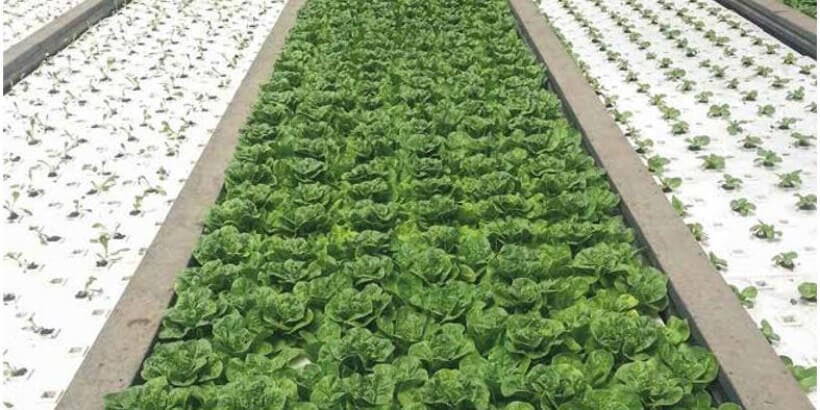This photograph showcases a well-organized agricultural field segmented into three distinct rows, bordered by gray cement barriers approximately 5 inches wide. The central row is densely packed with dark green, leafy vegetables, likely lettuce or cabbage, completely concealing the soil beneath. On either side, the left and right rows feature freshly planted smaller green plants, spaced generously apart and set against a white background that appears to be reflecting sunlight, suggesting the use of lawn paper or another reflective material. The entire setup reflects a meticulous and clean approach to crop cultivation.